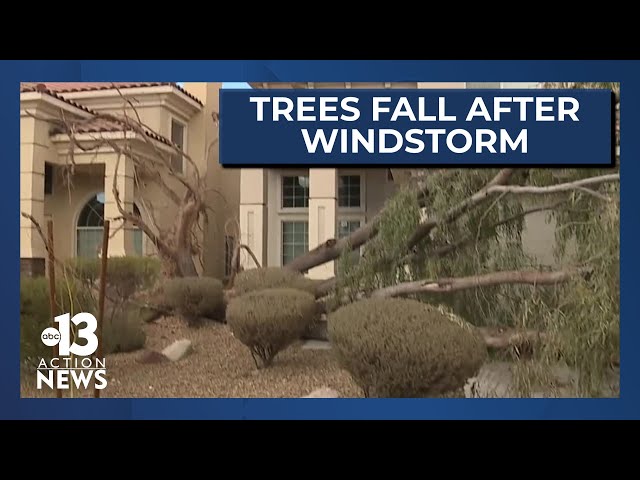This still shot from ABC 13 Action News, framed by a blue border against a black background, documents the aftermath of a windstorm in a ritzy neighborhood. The image, slightly washed out in color, features two adjacent mansions, one a tan Spanish-style structure with terracotta tiles and the other a paler tan. The central focus is on a large, uprooted tree lying across the front yard, seemingly obstructing the driveway and narrowly missing the houses. The broadcast includes a blue box with white text in the top right corner that reads, "trees fall after windstorm," emphasizing the hazardous yet apparently non-destructive incident. Despite some fallen branches and a broken tree stump, the houses, windows, and surrounding shrubs appear undamaged under clear blue skies, suggesting the aftermath of the storm is manageable.